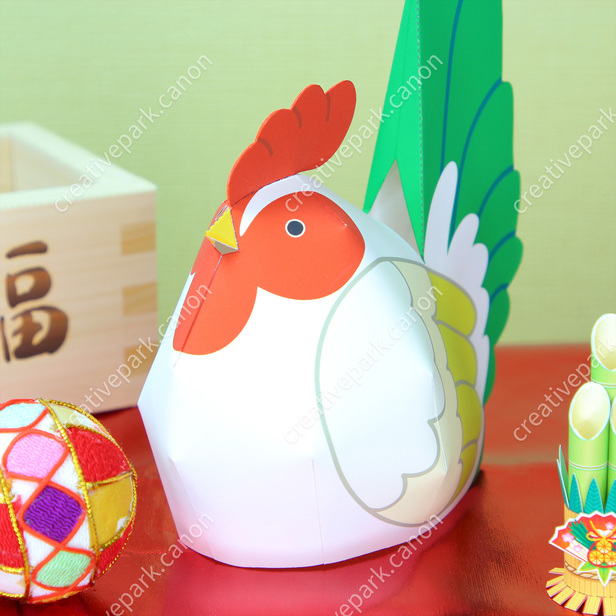This computer-generated image features a vibrant and whimsical scene centered around a distinctive paper chicken. The chicken, with a predominantly white body, displays intricate feather detailing—its wings transition from white through cream to yellow at the tips, while its tail feathers are a distinct green. The chicken's face is adorned with red markings around its yellow beak and black eyes, topped with a red feather.

Set against a soft green background wall, the chicken stands on an orange table. To the left of the chicken, there's an ornate, colorful fabric ball displaying a mix of purple, pink, aqua, red, and yellow diamond patterns. Beside the ball is a white, wooden square basket inscribed with Japanese or Chinese characters, contributing to the cultural motif of the scene. 

On the right side of the chicken are green paper bamboo shoots, accented with leaves that enhance the natural feel of the setting. Above the composition, the text "creativepark.canon" is subtly watermarked diagonally from the bottom left to the top right, indicating the source of this meticulously crafted digital artwork.